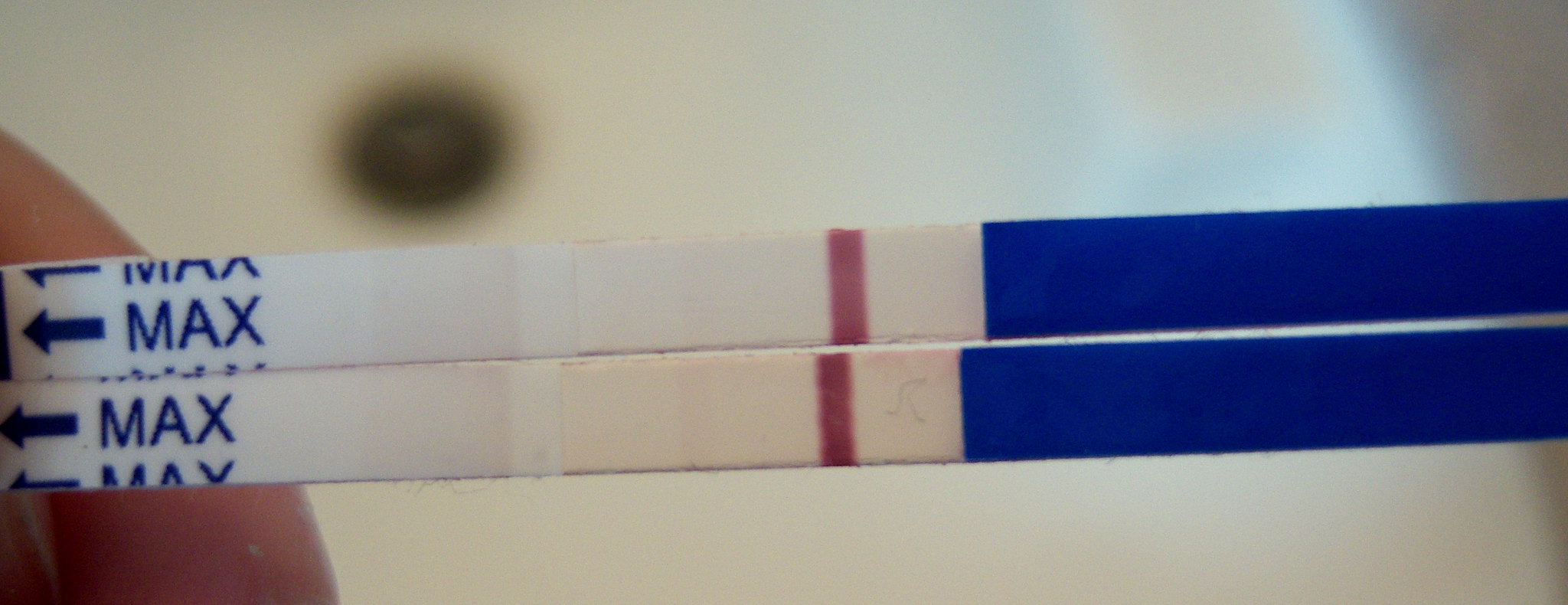This image features two rectangular testing strips, commonly referred to as paper pens. They are being held on the right side, revealing only a portion of the holder's finger, which appears to be Caucasian. The background displays a basin, suggesting it could be a bathtub or a large basin bowl, identifiable by a visible drainage area.

The testing strips themselves are long and skinny. On the left side of each strip, there is a blue arrow pointing to the left and the word "MAX" written twice. In the center of each strip, there is a very dark red line. The right portions of the strips are a deep blue color, with repeated blue writings and continuous dark blue lines. This detailed arrangement and color coding likely serve to indicate specific testing results.